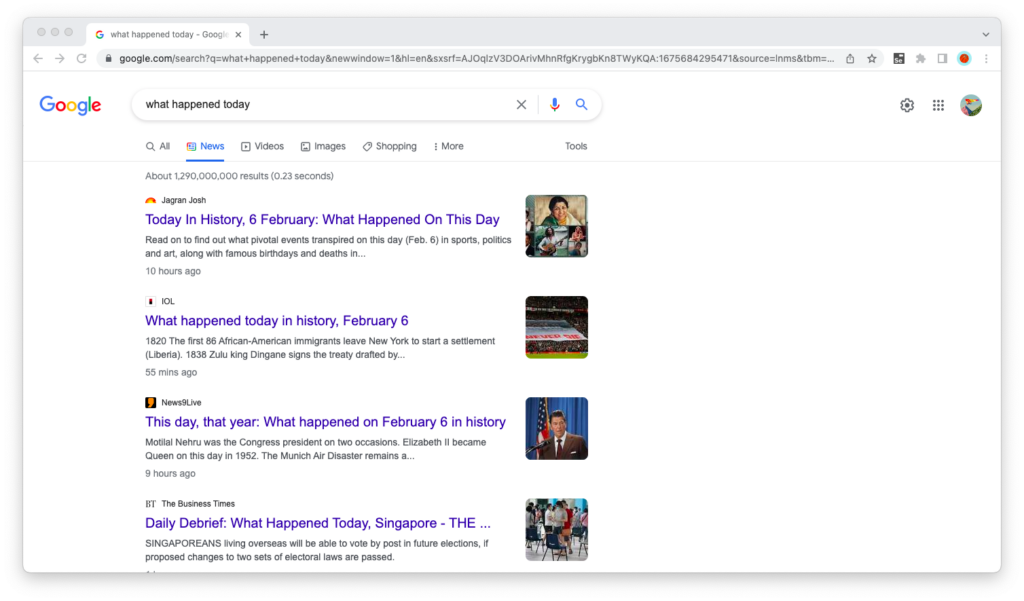Here's a detailed and cleaned-up caption:

---

The image is a screenshot of Google search results displayed within an unidentified browser, occupying the entire view. The browser interface is simple, featuring a light gray background at the top and a white-colored active tab. The tab shows the Google icon followed by the title "What happened today - Google." Adjacent to the tab title are the close button (X) and a plus sign (+) for opening new tabs.

Below the tab area is the address bar, which includes a padlock icon indicating a secure connection, followed by a long URL that starts with "https://www.google.com/search" and continues with a complex string of characters. The browser's navigation elements, such as back, forward, and refresh buttons, are also visible along with some browser extensions, suggesting it might be Google Chrome.

In the main body of the screen, the Google search page is visible. The user has searched for "what happened today." Below the search bar, the navigation tabs show various categories: "All," "News" (which is selected), "Videos," "Images," "Shopping," and more options available under "More" and "Tools."

The core content of the screenshot displays the news search results. The first result is from a website that appears to be named "Jagger and Josh," which features an article titled "Today in History, 6 February: What Happened on This Day?" accompanied by an image on the right and a snippet of text from the article, posted 10 hours ago. Below this, there are three additional news entries from different websites, each with corresponding images and preview text summaries. 

The entire search results section has a standard white background, suggesting that the user has not customized the Google theme. Additionally, a Google account avatar is visible in the top right corner of the window, indicating the user is signed in.

---

This caption provides a comprehensive and clear description of the image, capturing all relevant details in an organized manner.